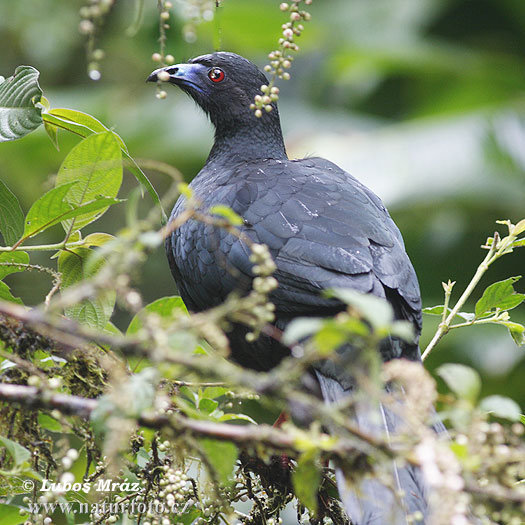This detailed wildlife photograph, taken by Lubos Mraz, captures an unusual black bird with a distinct profile and striking red eyes. Perched on a limb amidst green foliage, the bird features dark, almost blue-black feathers and a curved, black beak. It gazes to the left, seemingly oblivious to the photographer. The foreground showcases twigs, small flower buds, and the beginnings of berries, with a few white and pink flowers hanging gently above the bird. The background is softly lit and blurred, emphasizing the bird as the focal point. The image is softly lit with no distinct shadows, enhancing the serene atmosphere. The photographer's watermark is visible in the bottom left corner, reading "Lubos Mraz" along with the partially obscured website www.nature-22.cz.